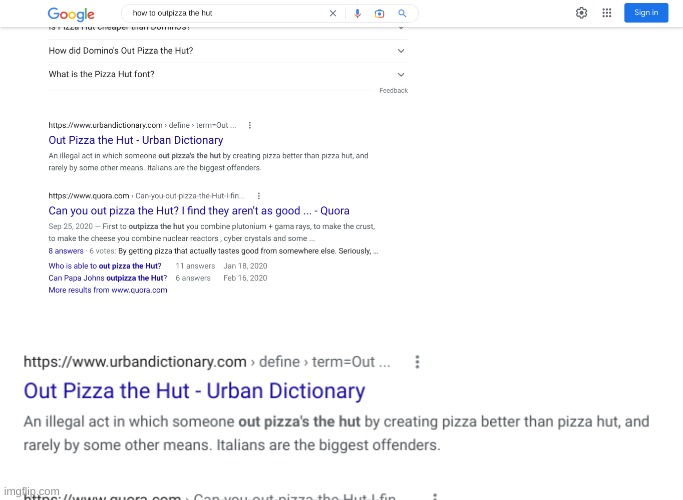The image depicts a Google search page with the query "how to outpizza the hut." The familiar Google logo is positioned in the upper left corner, while the "Sign in" option is visible in the upper right. The search results listed include various intriguing entries related to the query. The top result asks, "How to Domino's outpizza the hut?" following that, another entry questions, "What is the Pizza Hut font?" Below these, a link to Urban Dictionary appears with the term "outpizza the hut," and a subsequent result from Quora reads, "Can you outpizza the Hut? I find they aren't as good." Notably, the Urban Dictionary link is highlighted in larger text, making it more prominent among the search results.